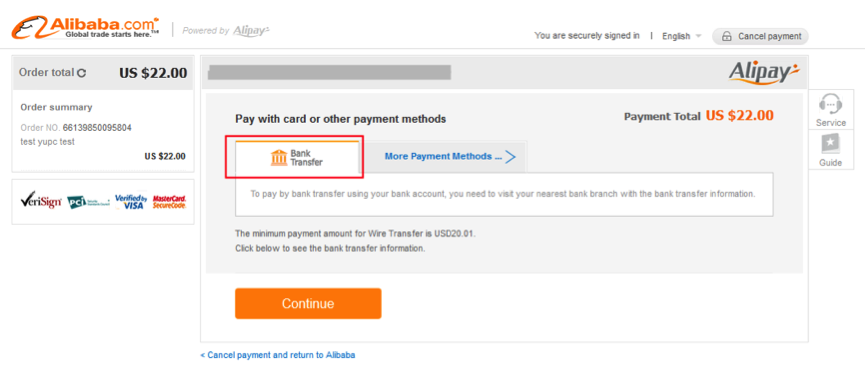The image is a detailed screenshot from the Alibaba.com website. The background is white, and in the upper left corner, the website name "alibaba.com" is prominently displayed. The word "Alibaba" is in bold orange font, while the ".com" is in a lighter orange and non-bold font. Beneath this, in a very small gray font, is the company slogan "Global Trade Starts Here." To the left of the text is the Alibaba logo, an orange design that somewhat resembles a question mark.

The page displayed pertains to Alipay, one of Alibaba's services, specifically for online payments akin to PayPal. The page layout includes a gray border. On the left side, it indicates the "Order Total: US $22" and beneath that, an "Order Summary" section with the order number and repeated total of "US $22.00".

In the center of the page, the order total "US $22" is highlighted in bold orange font immediately beneath the gray border. On the right side, the "Alipay" brand is written in gray font, with the dot above the letter 'I' and a dot at the tip of the letter 'Y' in orange, accompanied by a small, orange squiggly line underneath, adding a stylish touch to the logo.

Highlighted on the left side within a red rectangle is the text "Bank Transfer." To the right of this, in blue font, is the link "More Payment Methods," followed by a blue arrow, which suggests it's a clickable link.

At the very bottom of the screen, there is an orange rectangular "Continue" button with the word "Continue" in white font. Beneath this, in blue font, is the option to "Cancel Payment and Return to Alibaba," allowing the user to cancel the transaction if desired.